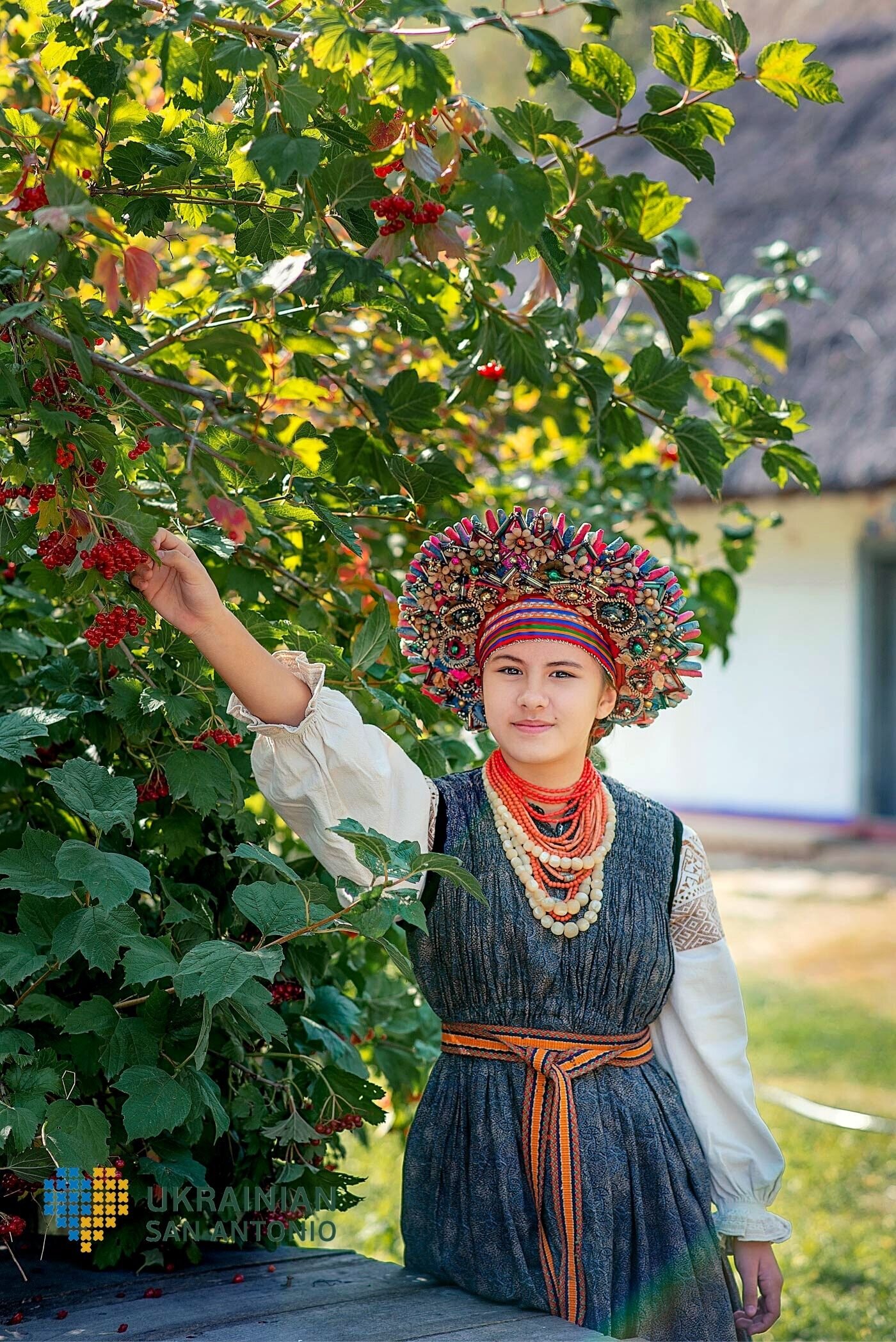In this vertical rectangular photograph, a young girl stands in a domestic garden setting, surrounded by elements that emphasize her traditional attire and the scene's cultural significance. She is positioned in front of a large bush or tree that is adorned with red berries, one arm raised as if to pick them. The backdrop shows a grassy area with a nearby table, and a white building featuring a gray roof appears in the background.

The girl wears a distinctive native costume—a dark blue jumper-style dress over a white puff-sleeve blouse with an orange and blue tie. Adorning her neck are numerous bright orange and white beaded necklaces, some of which resemble pearls. Her head is crowned with an elaborate, wide headdress that features a headband and an intricately detailed surface with bright colors, including pinks, blues, and golds, all concealing her hair beneath it.

She gazes directly at the camera, her face displaying a gentle smile. The bottom left of the photo bears the text "Ukrainian San Antonio," accompanied by a heart icon split into the blue and yellow colors of the Ukrainian flag, suggesting a cultural homage or connection to Ukraine.